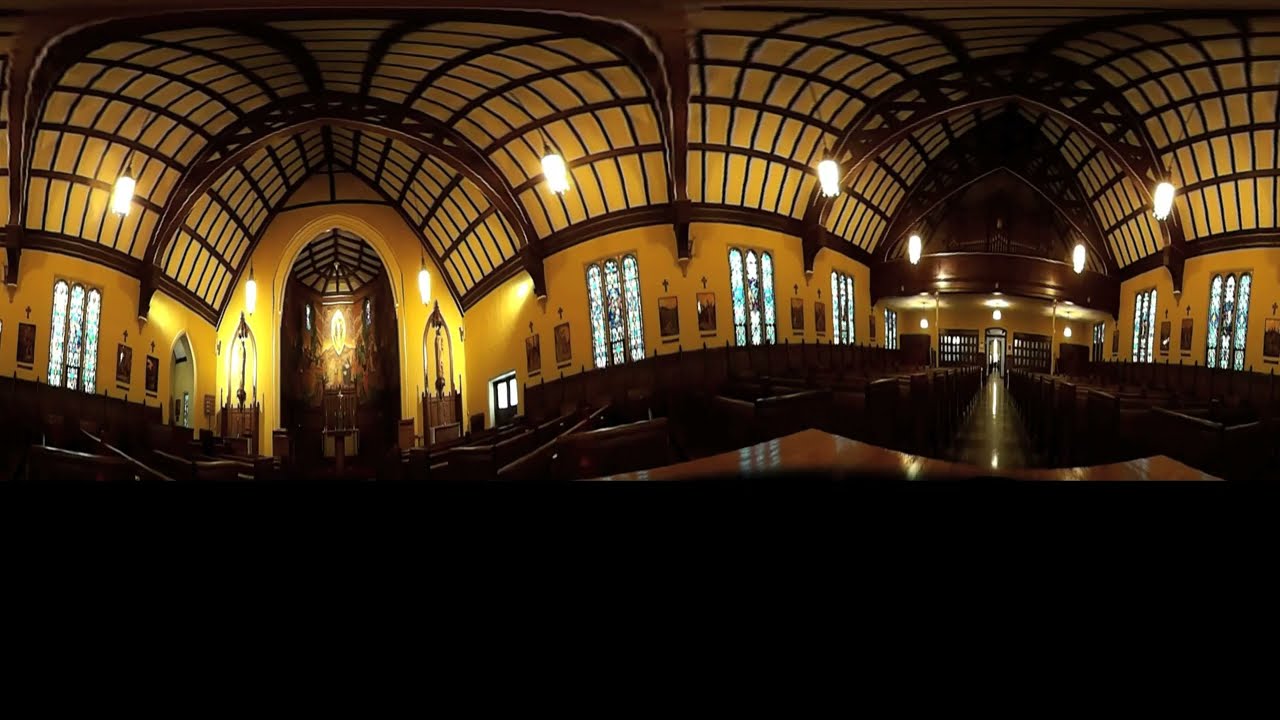The image is a detailed photograph capturing the interior of a massive cathedral church. Dominated by hues of yellow and brown, the scene showcases a distinguished blend of architectural beauty and religious elements. The floor and rows of pews stretching from left to right are primarily brown, creating a grounded, earthy atmosphere. The walls, illuminated by ambient lighting, radiate a warm yellow tone. 

Stained glass windows—colored in blue, brown, and white—adorn the church, adding a layer of intricate artistry. The ceiling, a mixture of light tan and deeper brown, features dark brown crisscross beams and archway beams, each decorated with subtle cutouts.

The photograph is taken from a side angle, capturing the altar on the left side where the priests would stand, framed by large archways and paintings. In the center and extending towards the back wall are numerous pews, enriching the scene with their symmetrical arrangement. On the right side, additional pews and a door leading to an exit are visible.

Above, hanging light fixtures contribute to the serene and meditative ambiance of the space. The top third of the image is primarily the ceiling with its detailed architecture, while stained glass windows line both sides of the church. The photograph, rectangular in shape, blends both sides of the church into one coherent, elegant composition showcasing its vast and serene interior.